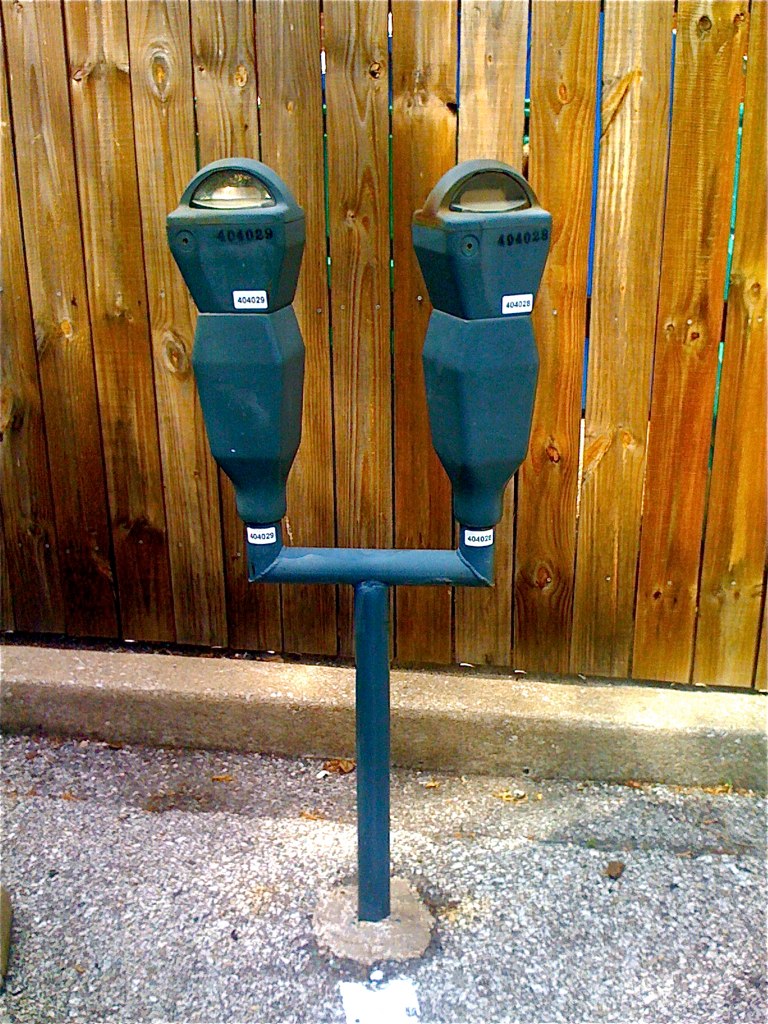The image showcases a pair of old-fashioned parking meters, mounted on a dark blue Y-shaped pole. These meters are connected at the top, each featuring a semi-circular dome with a transparent section beneath it. The numbers "494028" and "404029" are printed on white stickers attached to the meters, serving as their identification. The pole is securely anchored into the ground amid small rocks. The background consists of a light brown, unfinished wooden slat fence, situated behind a concrete curb. The setting includes an asphalt ground, adding to the aged, urban atmosphere of the scene.